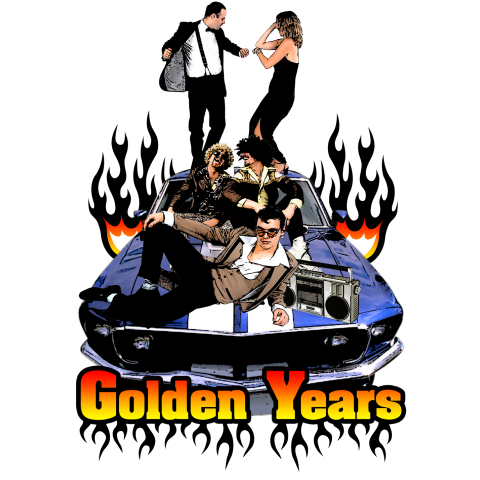The image, resembling a vibrant and nostalgic movie or event poster, features a vividly blue, Camaro-like vintage sporty car adorned with two thick white stripes running the length of its body. Leaning against the front of the car, a man dressed in 70s-style clothing—black pants, a fitted gray shirt, and a white-collared shirt—casually rests with his arm on a boombox, embodying a laid-back, cool persona. On the car’s roof, another man, clad in suspenders and a blazer, dances with a woman in a long black dress with a slit. Both the man and woman, who appears to be blonde, are captured mid-dance, facing each other in formal attire that evokes a timeless elegance. 

Adjacent to the windshield, two men are depicted in conversation, laughing and adding to the lively ambiance. The car's surroundings are framed by striking flames—predominantly black with red, yellow, and orange gradients—that enhance the retro and rebellious vibes of the scene. Below the car, the title "Golden Years" is prominently displayed in a font with a gradient effect from red to yellow, complemented by the same black flame motif underneath, solidifying the poster's aesthetic of a bygone yet golden era. The entire composition combines photographic and illustrative elements, creating a captivating and dynamic homage to vintage Americana and the vibrant spirit of the past.